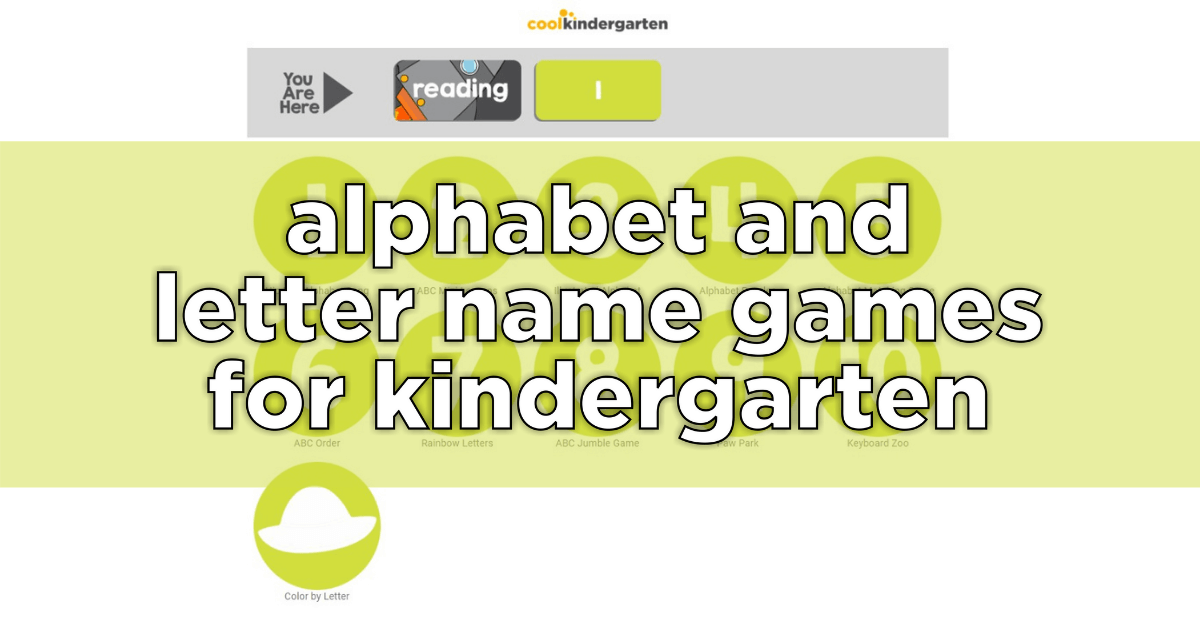The image showcases a carefully designed website titled "Cool Kindergarten" with "Cool" written in orange and "Kindergarten" in black. A small orange icon is cleverly positioned over the letter "L" in "Cool" and the letter "K" in "Kindergarten." Directly beneath this title, there's a gray navigation box with a message indicating the user's current location: "You are here," accompanied by an arrow pointing to a card-like graphic.

This graphic resembles a credit card and is shaded in various tones of gray. The word "Reading" is boldly inscribed in white across it, with a small blue dot positioned above the text. In the lower left-hand corner of this card, there are two orange blocks of different sizes, each featuring two orange circles. Adjacent to this is another card-like graphic, distinctively solid lime green, contrasting against the gray background, and displaying a prominent white number "1" in its center.

Below this header section lies a large, vibrant green box. Within this box are five circular icons, each one intended to represent letters, although the specifics are obscured by the superimposed text: "Alphabet and Letter Name Games for Kindergarten," written in white. Smaller, nearly indistinguishable print appears at the bottom of this green section, blending into the background.

Just below the large green box is another circle labeled "Color by Something," featuring a green background with a white hat icon in the middle. This element adds an educational and playful touch to the interface, suggesting activities or games related to color recognition or creativity.